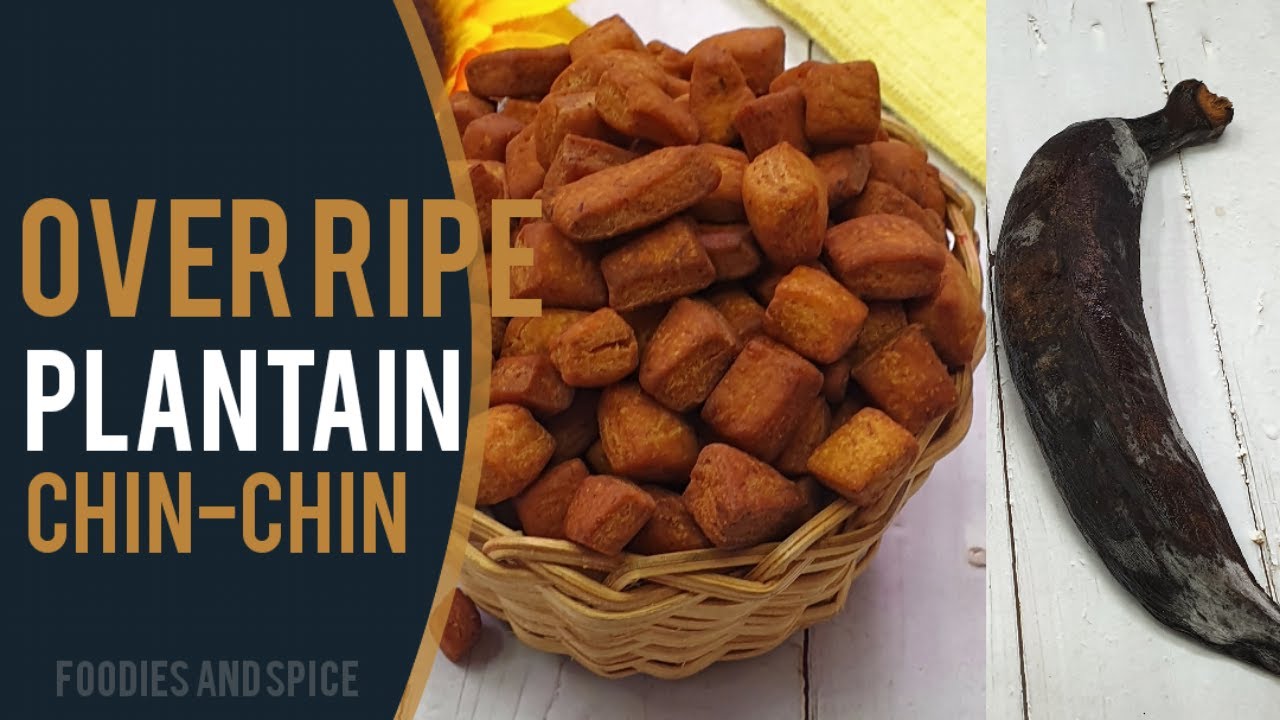This promotional image, likely for a blog post or food advertisement, features a striking and detailed arrangement centered around overripe plantain chinchin. The setting includes a white wooden table where a wicker basket brimming with reddish-brown, cube-shaped fried plantains, identified as chinchin, takes center stage. To the right of the basket lies an exceptionally ripe, black plantain peel, emphasizing the ingredient's maturity. On the left side of the image, a semi-circle in dark blue background features text in various colors: gold letters spell out "overripe," large white letters spell "plantain," and smaller brownish-gold letters say "chinchin." In the bottom left-hand corner, faint text reads "Foodies and Spice," unifying the promotional theme. The overall composition highlights the theme of utilizing overripe plantains to create delicious chinchin snacks.